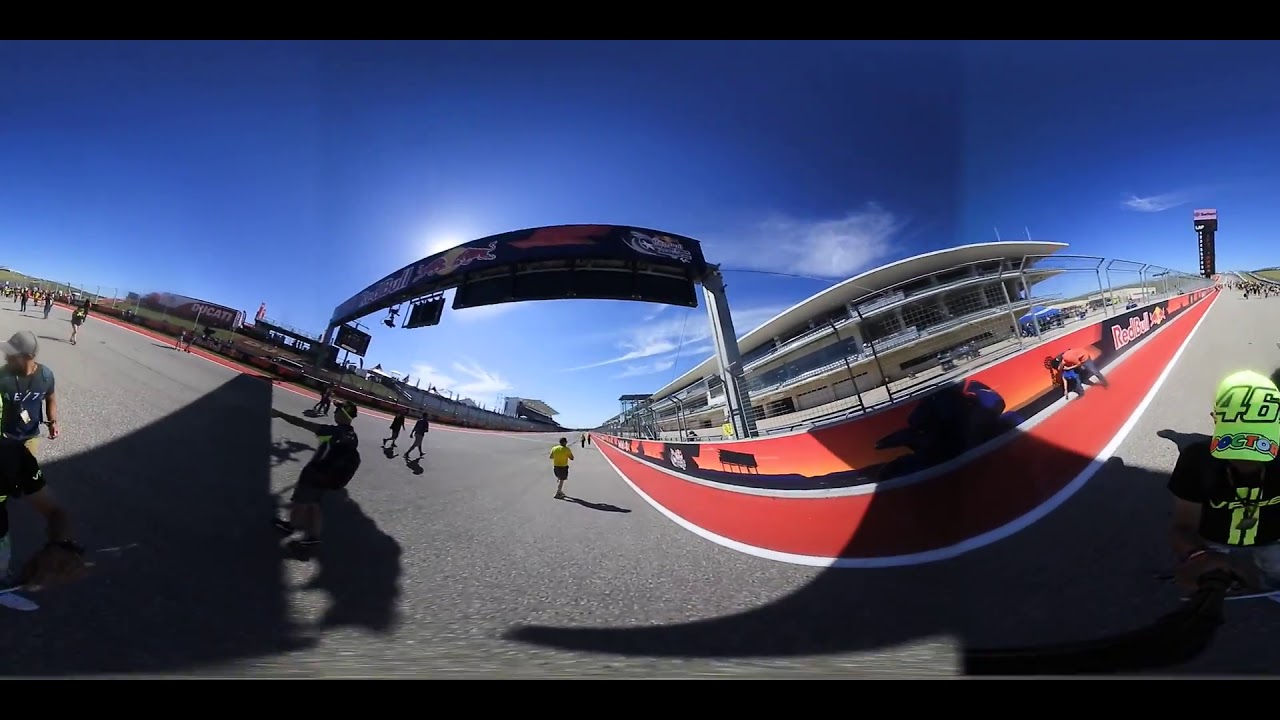This wide-angle, panoramic image of a racetrack captured with an extreme 180-degree fisheye lens showcases a busy scene on a sunny, late afternoon with a perfectly blue sky and distant clouds. The track features a pronounced start-finish line marked by a sign suspended between two poles. Bordering the track are distinct red and white lines leading up to a fence adorned with Red Bull branding. Behind the fence stands a circular, glass-front building topped with a white roof. On the track, a gentleman in a yellow shirt and black shorts is either walking or running towards the finish line, accompanied by several workers positioned on both sides of the track. A notable detail is a motorcycle numbered 46, possibly with a yellow wheel protector, located at the lower right corner of the image. In the background, a tower for results is prominently visible. The track's stands are noticed in the periphery, with people scattered around, either walking or running, adding to the vibrant scene. The sun, partially obscured by the overhead start-finish sign, casts a clear light, enriching the detailed and dynamic atmosphere of the racetrack.